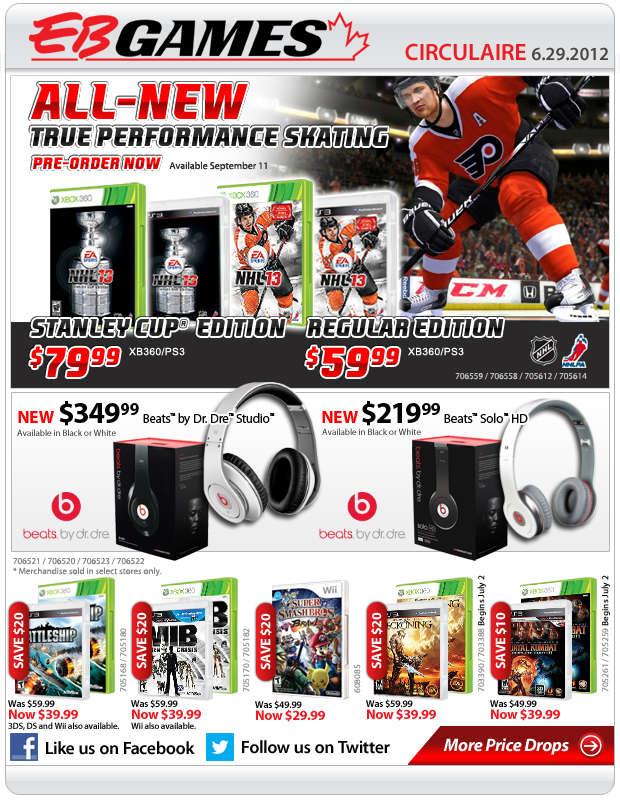This vibrant digital flyer from EB Games boasts a sleek white background accented by bold red and black text. In the upper areas of the flyer, the EB Games logo is prominently displayed in the upper left corner, while the top right corner announces "Circular" in vivid red text with the date "6-29-2012".

Dominating the center of the flyer, a compelling advertisement for EA Games' NHL 13—Stanley Cup Edition and Regular Edition—captures attention with its promotional bold typography and visuals. This section reveals that the special Stanley Cup Edition is priced at $79.99, whereas the Regular Edition is available for $59.99. Endorsements from both the NHL and potentially the NHLPA lend official recognition to the game. A thrilling in-game screenshot is placed on the right side, adding visual excitement to the promotion.

Below, a highlight section dedicated to high-end Beats by Dr. Dre headphones showcases two models: Beats Studio priced at $349.99 and Beats Solo HD at $219.99. Each model is presented with a picture of both the product and its packaging, emphasizing its premium quality.

The flyer also features a section at the bottom with various video games that have received significant price drops. Titles such as Battleship, Men in Black, Super Smash Bros. Brawl for Wii, Reckoning, and Mortal Kombat are now available for $29.99 or $39.99, reduced from their original prices of $49.99 or $59.99. 

The flyer concludes with a call to action, encouraging readers to engage with EB Games on social media by liking their Facebook page and following them on Twitter, along with hints at additional price reductions.